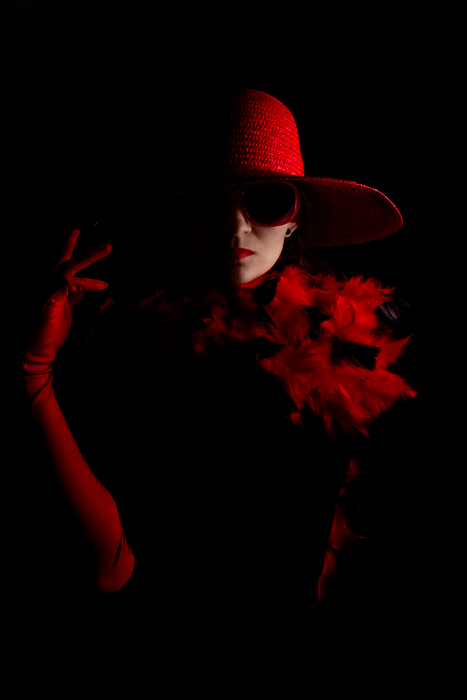The image presents a striking portrait of a Caucasian woman against a completely black background, with dramatic lighting highlighting only the right side of her figure. She appears to be partially engulfed in shadow, creating a stark contrast between light and dark. The woman is adorned in a vibrant red ensemble that includes a stylish sun hat and matching sunglasses with black accents. Her lips are painted a vivid red, complementing the red earrings she is wearing. Draped over her shoulders is a red feathery jacket or shirt, which adds texture and complexity to her attire. On her right arm, she is wearing a long red sleeve that resembles a glove extending up her arm. Feathers cascade down her left side, although the darkness obscures details below her torso, creating an intriguing illusion where only half of her face and a single hand are clearly visible. Despite the obscured elements, the image exudes an aura of mystery and elegance, drawing focus to the vivid red details against the pitch-black background.